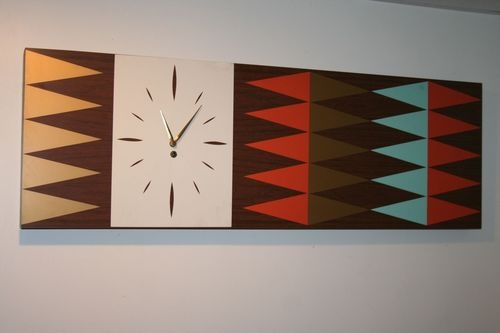The image presents a horizontally rectangular frame showcasing an off-white wall adorned with a distinctive clock. The clock itself occupies a section in the center of the frame and features an off-white face with gold-colored hands and markings, which include simple bars in lieu of traditional numbers. 

Flanking the clock face are multiple vertically aligned rectangular sections that resemble a backgammon board design. On the left side of the clock, there are yellow triangles pointing towards the right interspersed with brown rectangles directed towards the left. To the right of the clock, this design continues with additional sections featuring a mix of brown, red, blue, and red triangles and rectangles, maintaining the backgammon pattern aesthetic.

The clock, positioned centrally within the creatively segmented wall frame, stands out with its minimalist design, highlighted by the contrasting decorative patterns on either side, making it a striking element in the composition.